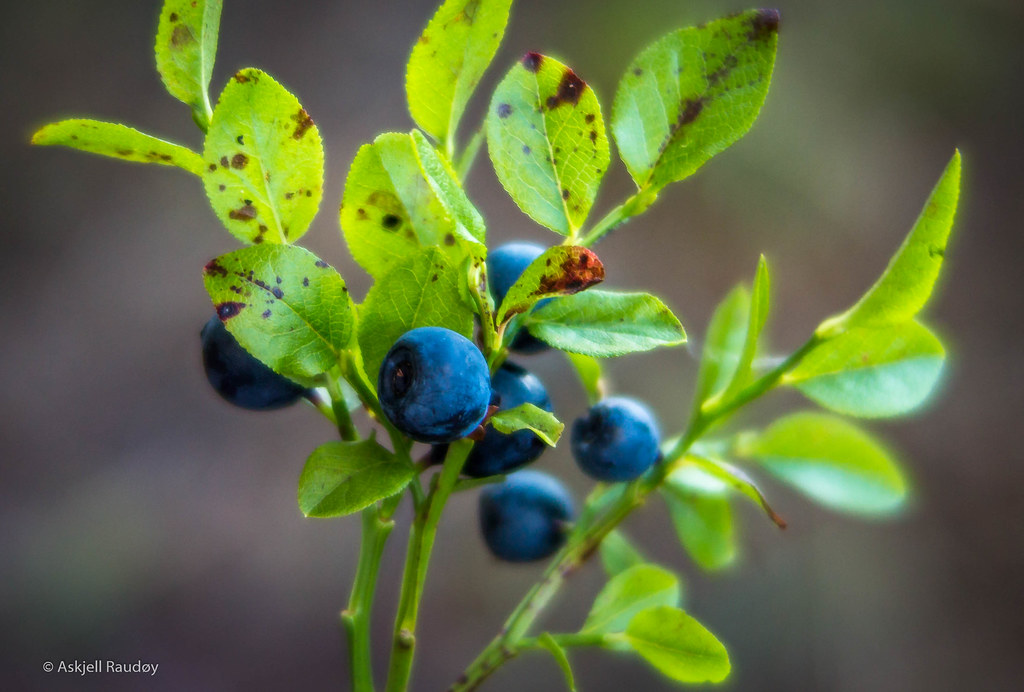This vibrant outdoor color photograph captures a close-up of a blueberry plant, its vivid green leaves sprouting from thin stalks. Some leaves feature reddish-brown splotches, adding character to the lush foliage. The plant proudly bears six ripe blueberries, with one prominent, crisp, and vividly blue berry at the center, while the other five blend softly into the artistically blurred background. The rest of the image is obscured by a beautiful bokeh effect, drawing all attention to the detail of the blueberry plant. In the lower left corner, there's a discreet copyright mark, crediting the photo to "Ask Gel Roddy" or "Ask Joe Raudoy."